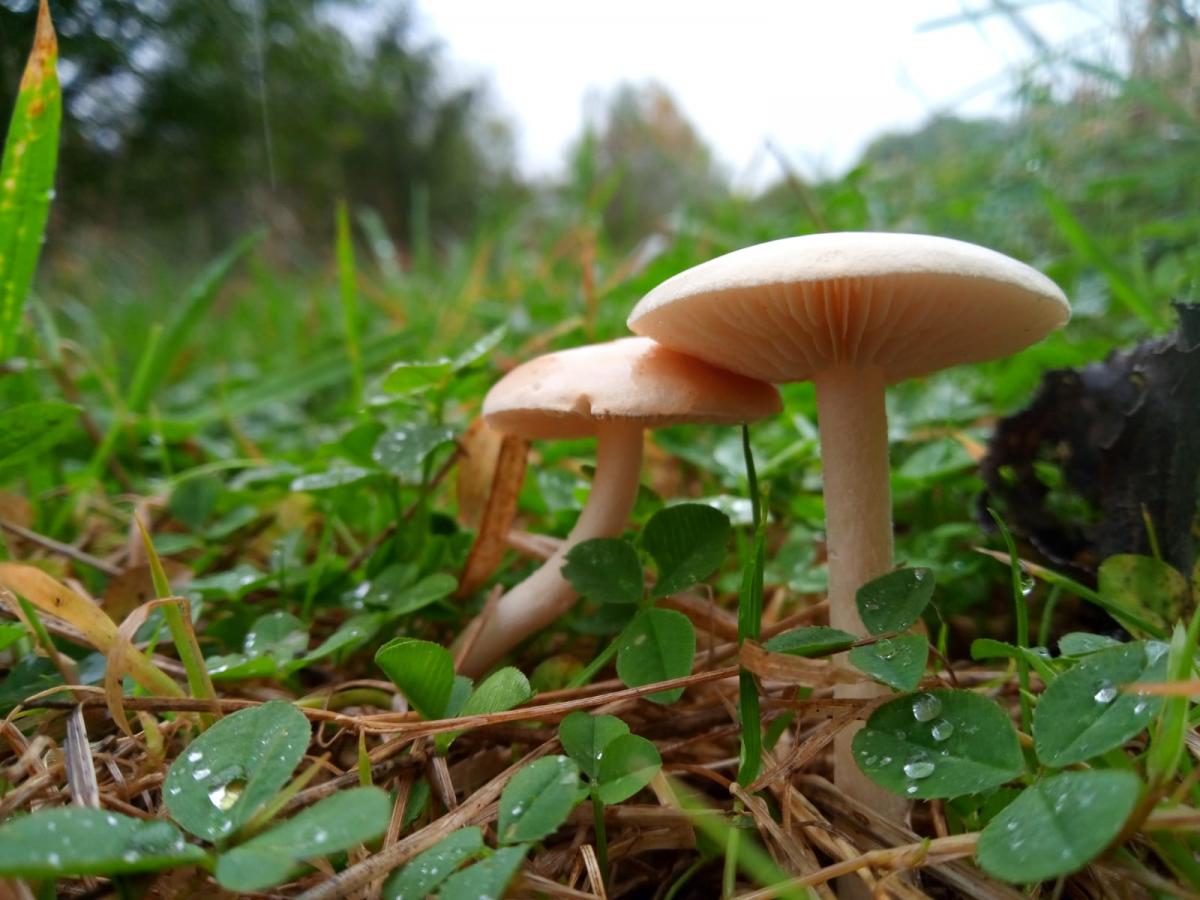This image captures a serene, close-up scene of two light pinkish-beige mushrooms standing amidst a mix of green and brown grass. Taken at ground level in a vertical rectangular frame, the focus is on the mushrooms, which are positioned slightly off to the left. The mushroom on the left leans into the one on the right, adding a sense of connection between the two, while the right mushroom stands straight, both featuring cylindrical stems topped with disc-like caps whose edges hang slightly downwards. The background subtly features a blurred blue sky and green trees, enhancing the peaceful atmosphere. Adding to the tranquility are green clover-like leaves with droplets of dew, symbolizing the gentle touch of Mother Nature at work.